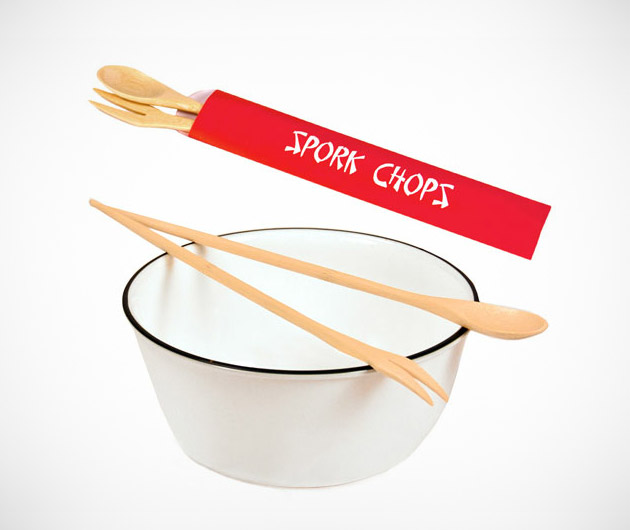The image features a pristine, white background showcasing a minimalist scene centered around a white, Asian-style bowl with a distinctive black trim. Resting diagonally across the top of the bowl are two wooden utensils—a spoon and a fork. Above the bowl, seemingly floating, is a red paper package labeled "Spork Chops" in bold white letters. This package contains an identical set of wooden utensils, partially visible as they extend out from the packaging. The composition is clean, with no shadows, emphasizing the contrast between the white background and the red packaging, making the "Spork Chops" product the focal point of the image.